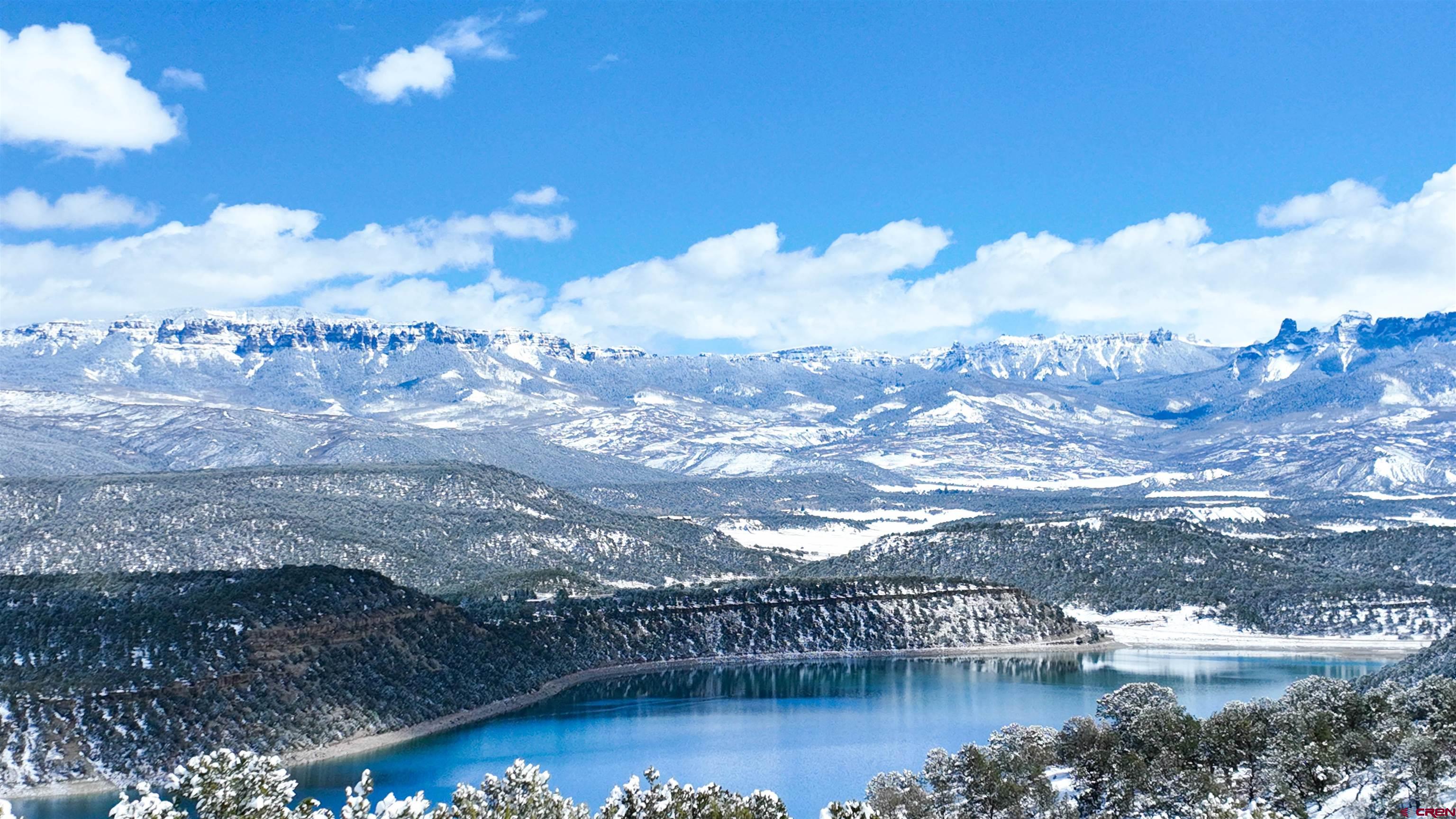The image captures an awe-inspiring winter scene in an outdoor mountainous region. Dominating the landscape are majestic snow-covered mountains, which extend from the central background to both the left and right sides of the image. The clear blue sky, adorned with wisps of white clouds, frames the peaks beautifully. In the foreground, a pristine, light blue lake reflects darker shadows, suggesting its clarity and depth. This pure, crystalline water, exhibiting hints of green, sets off the contrasting rich green trees scattered around the lake’s edge, some dusted lightly with snow. The middle ground showcases sloped cliffs adorned with trees, snow, and striking rock formations, adding to the rugged beauty of the scenery. As the gaze moves further back, the snow becomes more predominant, covering the terrain extensively. The image overall presents a harmonious blend of natural elements, capturing the serene yet striking beauty of a winter landscape.